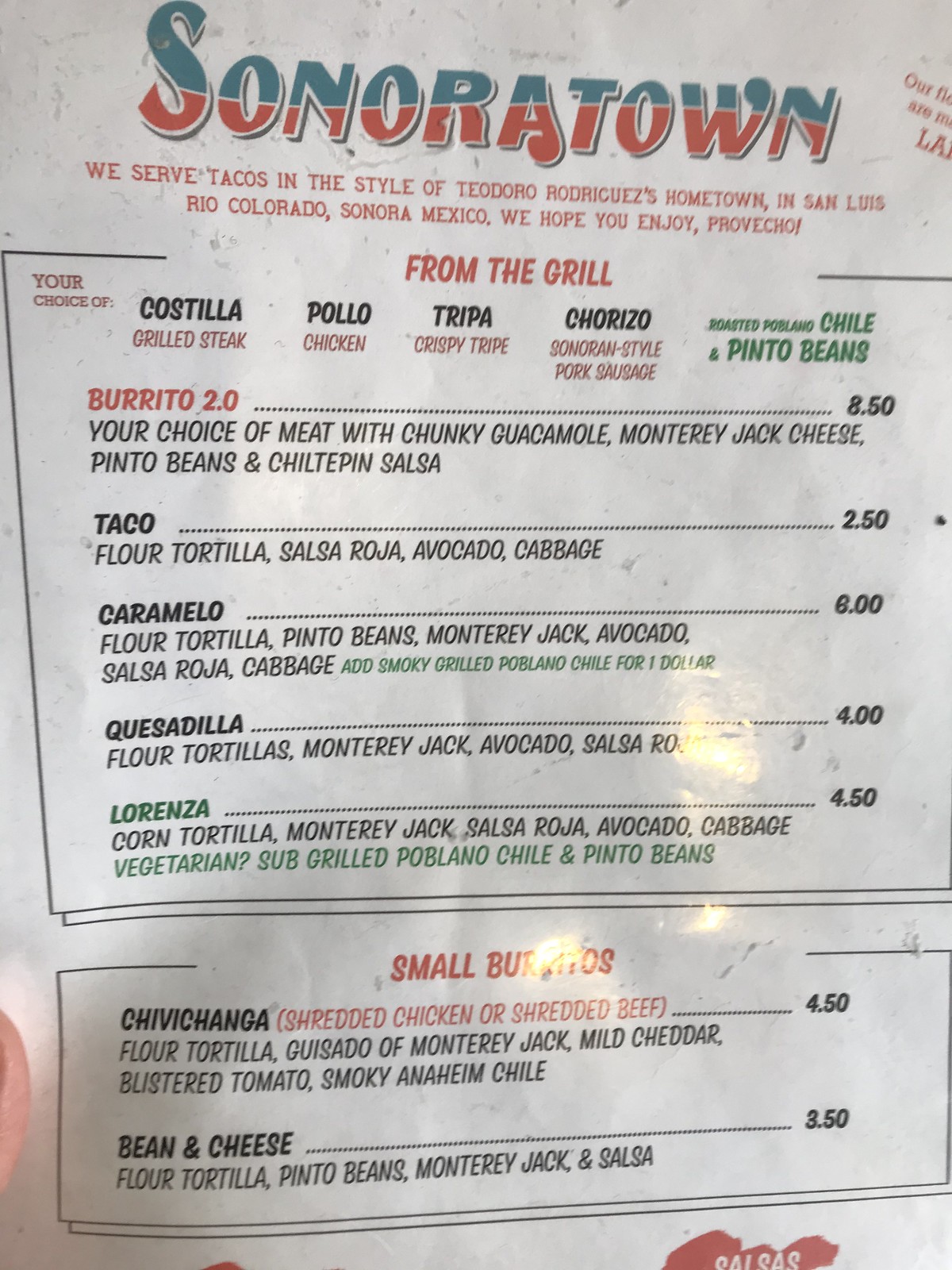The menu, printed on white paper, prominently displays "Sonoratown" at the top in a striking mix of blue and red lettering. Below that, in red letters, it reads, "We serve tacos in the style of Tadora Rodriguez's hometown in San Luis Río Colorado, Sonora, Mexico. We hope you enjoy, por favor." A black border frames the menu, adding a touch of elegance.

The section titled "From the Grill" is highlighted in red, followed by "your choice of" in black letters:
- **Costillo:** Grilled steak (red letters)
- **Pollo:** Chicken (red letters)
- **Tripa:** Crispy tripe (red letters)
- **Carrizo:** Sonora-style pork sausage (red letters)
- **Chili and Pinto Beans:** (green letters)

Menu options include:
- **Burrito #2:** Your choice of meat, chunky guacamole, Monterey Jack cheese, pinto beans, and chilled pen salsa.
- **Taco:** Flour tortilla with salsa roja, avocado, and cabbage.
- **Caramelo**
- **Quesadilla**
- **Lorenza**
- **Chimichanga**
- **Beef and Cheese**

Each option is thoughtfully crafted to reflect the authentic flavors of Sonora, Mexico.